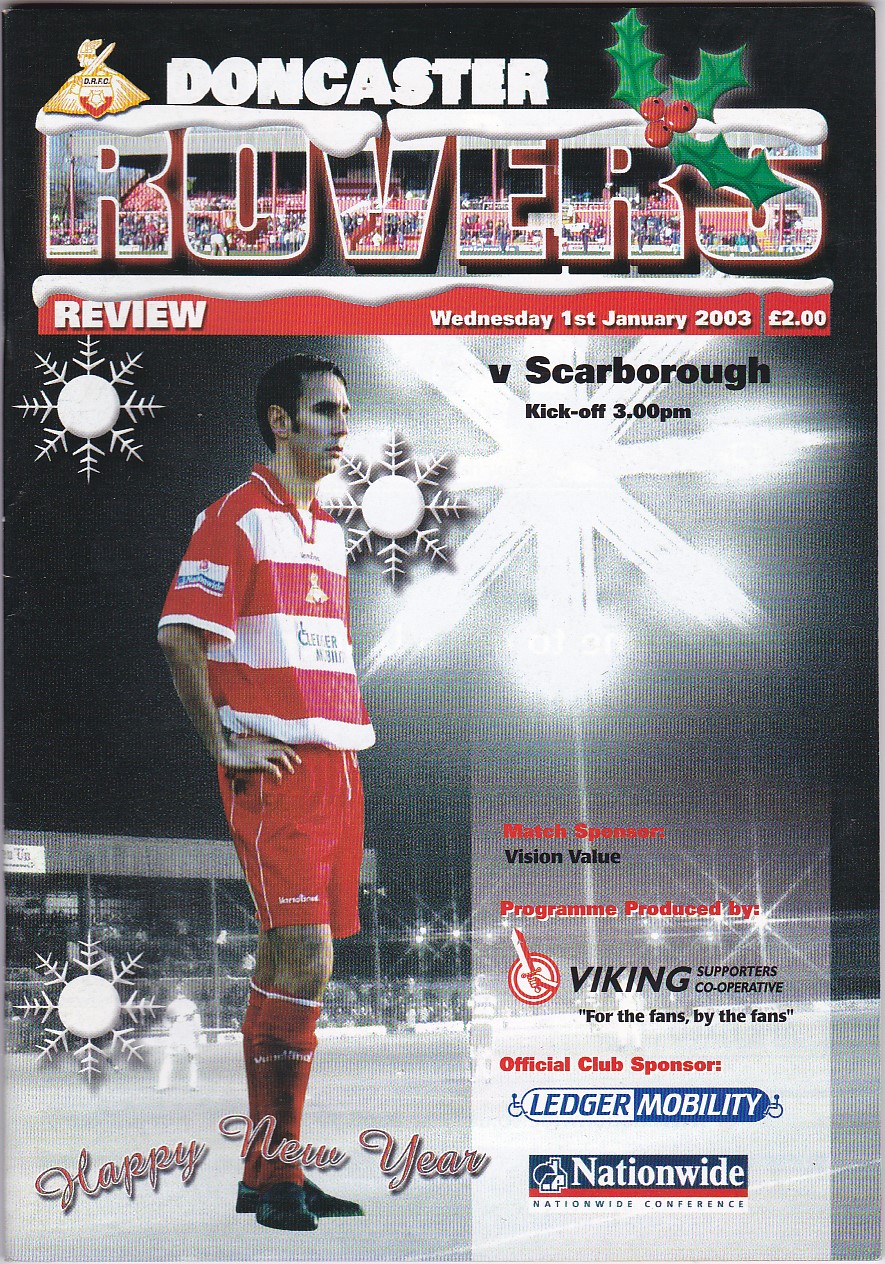The cover of the sports magazine, primarily focusing on the Doncaster Rovers, showcases a tall rectangular design. Dominating the backdrop is a stark black and white photograph of a soccer field, resembling a turf field, bordered in the distance by a large gate and a sizable seating area on the left side, illuminated by several bright lights. The top portion of the image transitions into solid black, contrasting the detailed scene below.

On the right side of the cover, a large white snowflake drawing is prominently displayed. Meanwhile, on the left, a cut-out picture features a player sporting the Doncaster Rovers uniform: a red and white striped jersey, red shorts, and red socks paired with black shoes. This player stands out vibrantly against the monochrome background, seemingly placed on a snowy field.

At the top of the magazine, the title "Doncaster Rovers" stands out, with "Doncaster" in white font and "ROVERS" displaying picturesque scenes within the letters, embellished with a layer of snow on top. Below this, it reads: "REVIEW, Wednesday 1st, January 2003, £2" in white text set against a red background, also topped with snow.

Additional text on the cover includes "SNOWQUAKE" in white against the black backdrop, advertising the upcoming Scarborough kickoff at 3pm. The player’s feet are adorned with the phrase "HAPPY NEW YEAR" in red letters. Nearby, it reads "MATCH SPONSOR" in red, followed by "VISION VALUE" in black. Further down, the cover notes that the program is "PRODUCED BY" the "VIKING SUPPORTERS COOPERATIVE," identified by a logo of a fist holding a sword, and the taglines "FOR THE FANS, BY THE FANS." The official club sponsor "LEDGER MOBILITY," is also highlighted, with "LEDGER" in blue on a white background and "MOBILITY" in white on a blue background, flanked by images of people in wheelchairs facing inward and "NATIONWIDE" in white on a blue background with a small house and tree icon, followed by "CONFIDENCE" in black or blue on a white background.

The intricate details and festive imagery make this program cover a visually engaging piece for supporters of the Doncaster Rovers.